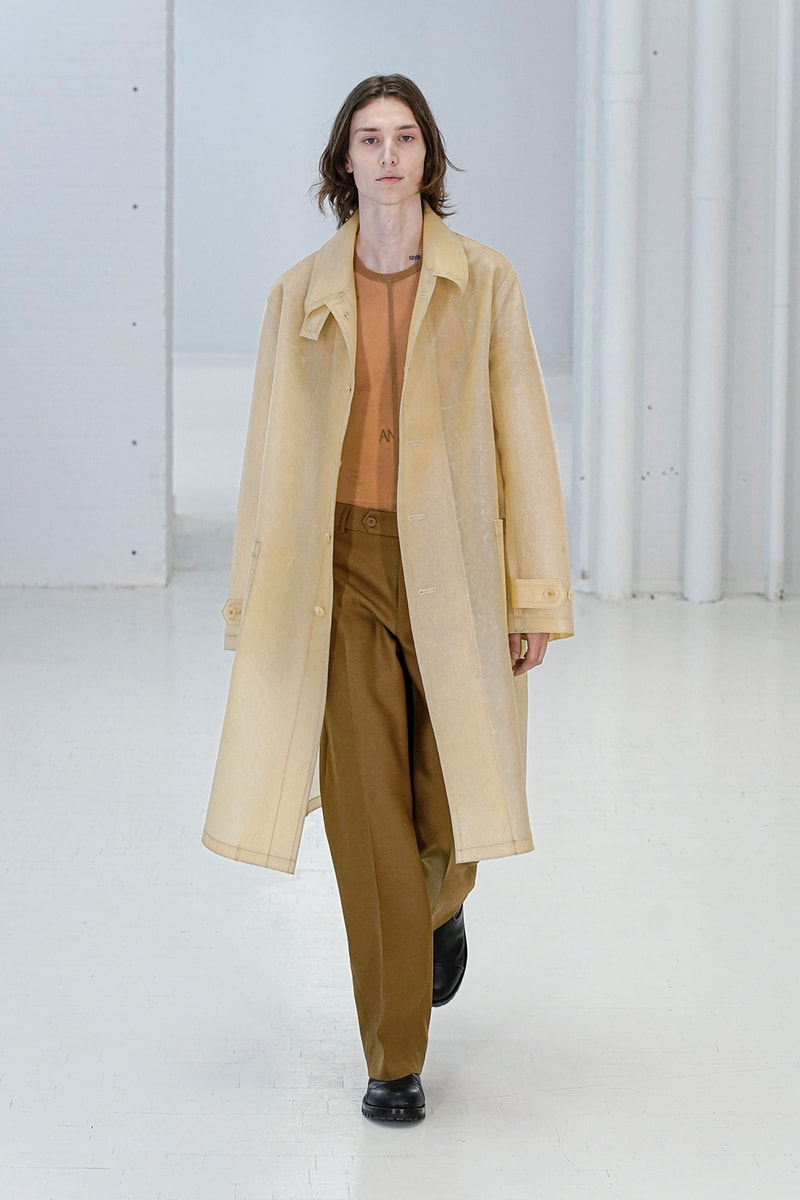The photo depicts a tall, slender model with shoulder-length dark brown hair, walking mid-stride directly toward the camera on a white catwalk. The model, with pointed features and a stern, emotionless expression, is wearing black shoes, brown pants, a see-through orange top, and an undone long tan raincoat-like garment. The model's right leg is forward while the left leg is behind, suggesting motion. The background is entirely white, giving an impression of a minimalist runway setting. Their arms are straight and relaxed by their sides, and no accessories are visible. The model exudes a professional runway demeanor, exhibiting the attire chosen by the designer.